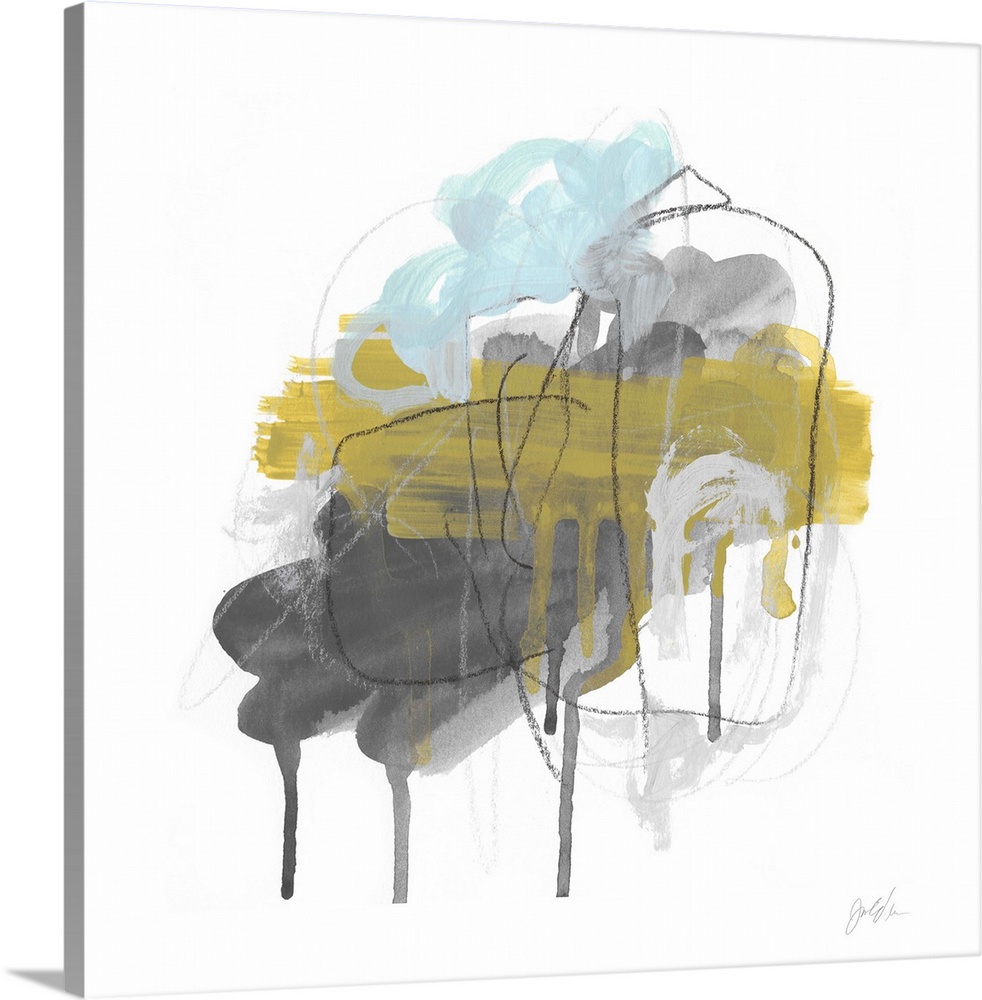This abstract painting, showcased on a square white canvas, features a captivating blend of mixed media elements and a variety of colors. The canvas has a visible gray side, which adds dimension, and is angled slightly towards the right. Dominated by a palette of gray, black, yellow, gold, and teal, the artwork boasts multiple layers that contribute to its intricate texture. At the base, gray paint strokes appear to have dripped with water, creating a dynamic background. Over this, splashes of yellow paint add vibrancy, accompanied by a horizontal stroke of muddy gold that also drips slightly. Blue clouds float atop, bringing a serene contrast to the composition. Black lines and crayon scribbles in both gray and black intertwine across the piece, including a black rectangle-like shape on the left. The painting is punctuated by a fine point pen signature in black script found in the lower right corner, with a discernible 'J'. This meticulous layering and the interplay of colors and textures make the painting a visually stimulating piece of abstract art.